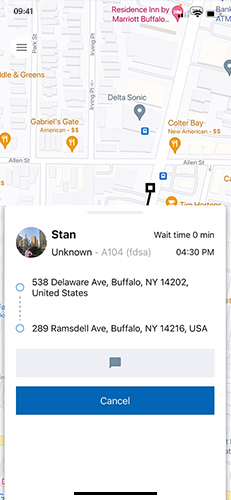The image showcases a digital map with a detailed route and relevant information overlaid. A posting by a user named Stan, whose profile picture suggests he is a Caucasian male (though the image is quite small and grainy), is prominently featured. The caption indicates that Stan's status is "unknown" and his wait time is listed as zero minutes, hinting that he might be an Uber driver or similar service provider.

The journey details are specified: either starting from or heading to 538 Delaware Avenue, Buffalo, New York, with the other end of the route being Ramsdale Avenue, Buffalo, New York. The exact direction of travel is unspecified. A blue flag icon is displayed inside a gray box, with a blue 'Cancel' button below it.

The map presents a green pin marking the key locations and depicts various landmarks along the route, such as the Residence Inn by Marriott and other notable spots in the vicinity. Despite the detailed map and route information, there is no additional contact information for Stan beyond his "unknown" status and the current wait time.